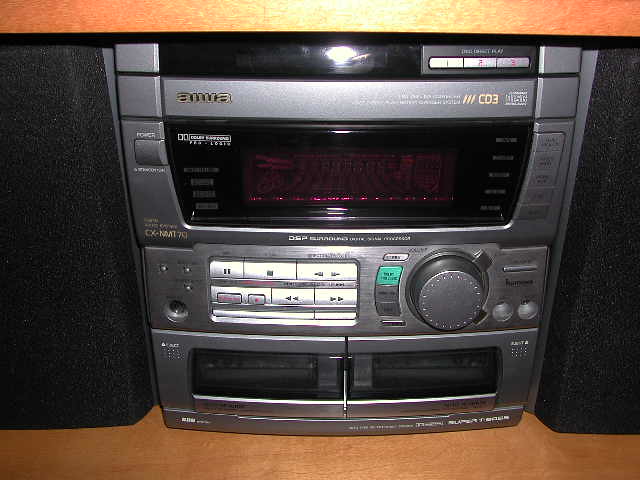This image features a close-up of an AIWA branded stereo system, placed on a light brown wooden shelf. The setup includes two large black speakers on either side of the central unit, with the characteristic fuzzy black grills partially exposing the silver edges of the speakers.

The main stereo unit in the center is divided into several sections. At the top, there is a compartment for CDs accompanied by three silver buttons. Below this section, there is a black, inactive display screen bordered in silver. The brand name 'AIWA' is prominently displayed toward the top left of this screen. Below the display, there are several control buttons including play, pause, stop, and rewind on the left side, and a large circular volume knob on the right, accompanied by two headphone ports.

The bottom section of the stereo features two silver-colored cassette tape decks positioned side by side. The power button is located on the left side of the unit, and the model number 'CXMT-70' is indicated as well. The overall aesthetic includes brown trim visible across the top of the shelf, emphasizing the vintage look of this multifunctional entertainment system.